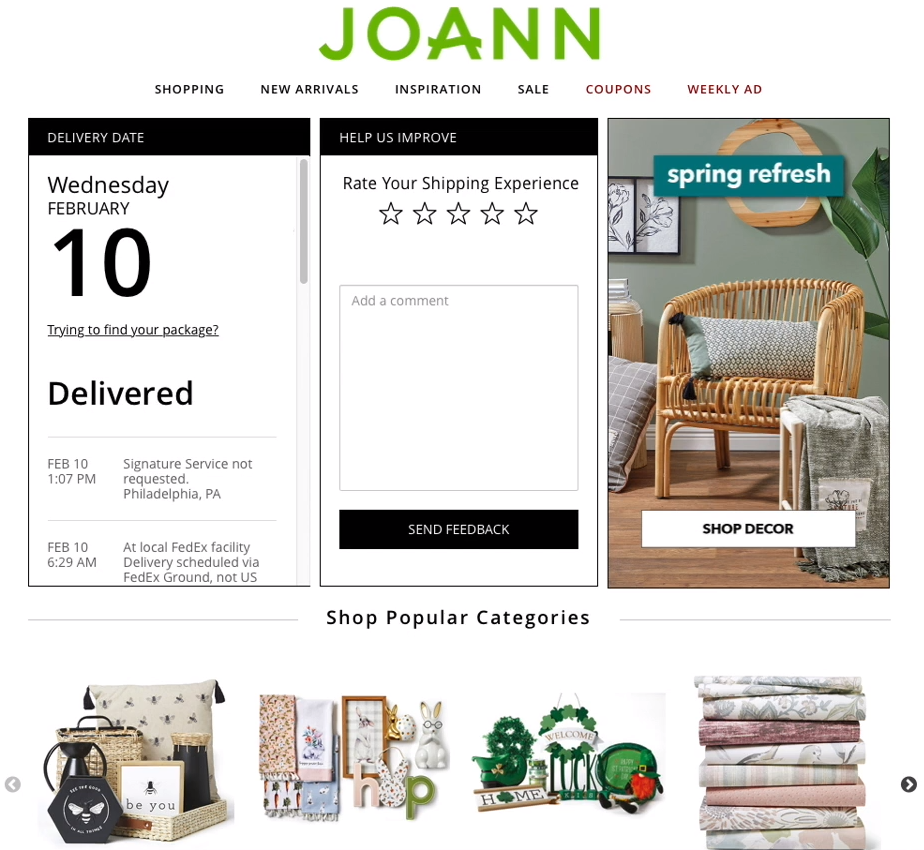The image shows a vibrant and detailed welcome page for Joanne's Home Décor Shop. 

**At the top of the page:**
- The name "Joanne" is prominently displayed in bold green letters, marking the branding for the Home Décor Shop.
- Directly below it, navigation options are enlisted: "Shopping," "New Arrivals," "Inspiration," "Sale," "Coupons" (in red text), and "Weekly Ad" (also in red text).

**In the next row:**
- On the far left, inside a black box, the text reads "Delivery Date" with the specific date "Wednesday, February 10th" mentioned below.
- Underneath this, there's the question "Trying to Find Your Package?" which is underlined, followed by the word "Delivered."

**To the right side:**
- Another long box contains the text "Help Us Improve: Rate Your Shipping Experience," with five adjacent empty stars for rating.
- Further right, a green box highlights "Spring Refresh," showcasing an attractive scene with a mirror on a wall, a picture, a wicker chair with a pillow, and below that, another box labeled "Shop Décor."

**At the bottom:**
- The section "Shop Popular Categories" is visually represented. 
  - On the far left, an image shows a wooden tray holding a white pillow decorated with black bumblebee prints, accompanied by a woven basket.
  - To the right, hand towels are displayed alongside a sign reading "Hop" and a little bunny figurine wearing glasses.
  - Finally, on the far right, stacks of towels or sheets in various shades of pink, white, and gray are neatly arranged.

The page overall offers a rich, organized, and inviting layout, guiding customers through several categories and promotional highlights.